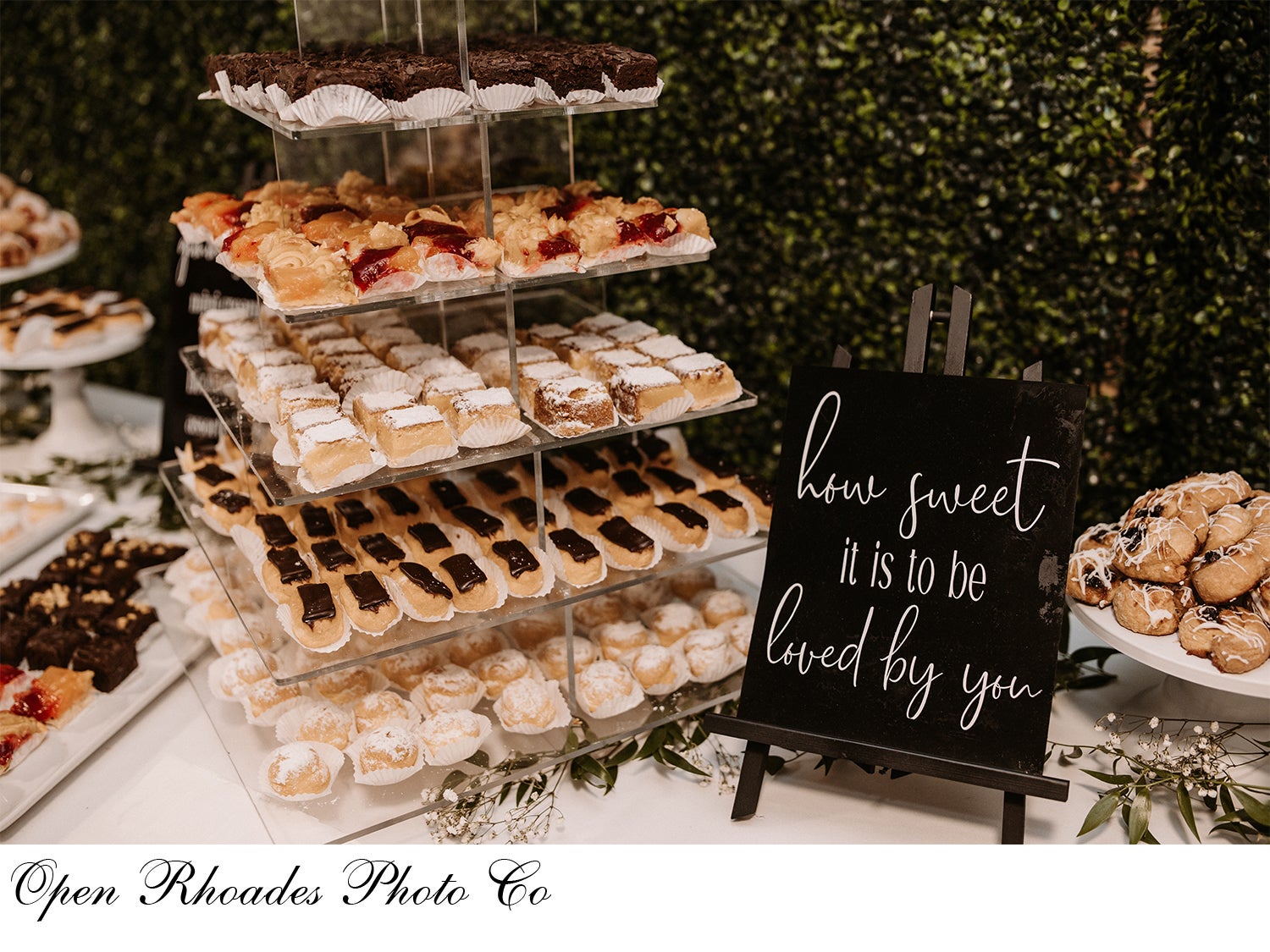In this photograph, an elegantly decorated table is adorned with a stunning array of desserts, perfect for an event like a wedding. The centerpiece is a five-tiered stand displaying an assortment of delectable treats, each nestled in its own fluted paper holder. The top level features bite-sized brownies, while other levels showcase mini eclairs, jam cakes, powder sugar cakes, and more unique pastries. To the right of this multi-level stand is another tray, possibly holding Danish pastries. Additional trays of fudge and assorted pastries are arranged to the left. All of this is set against a beautiful backdrop of an ivy-covered green wall, suggesting an outdoor setting. A black sign on a black easel, adorned with the words "How sweet it is to be loved by you" in white cursive font, adds a charming touch to the scene. The table itself is draped with a white tablecloth, and in the bottom left corner, the watermark "Open Roads Photo Co." is visible.